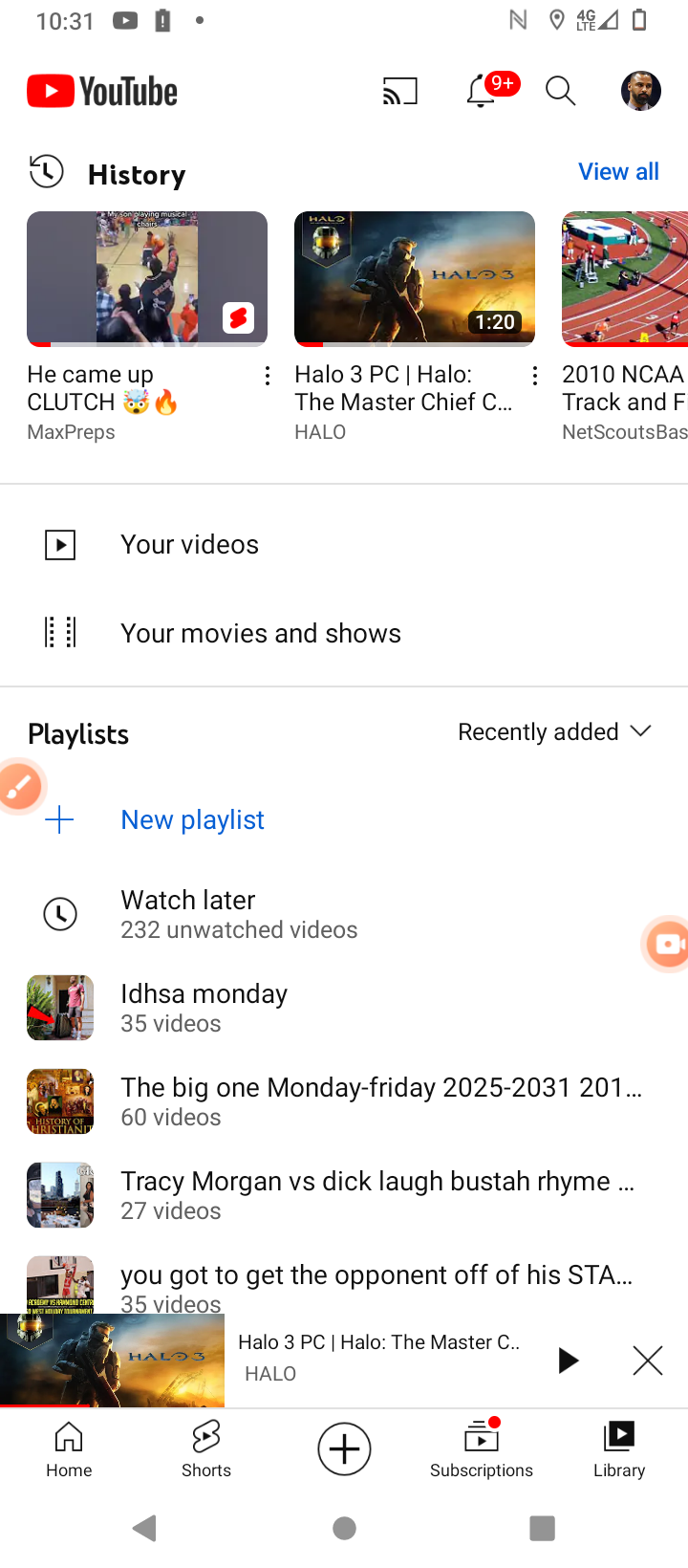The image is a clear screenshot of the YouTube app interface on a mobile phone. The phone's status bar at the top of the screen includes familiar icons such as the battery meter, clock, and signal strength indicator. Below this, the YouTube app header is prominently displayed, featuring the red YouTube logo and the title "YouTube."

The primary content of the screenshot showcases the user's watch history, with thumbnails and titles for various videos they have recently viewed. Among these, there appear to be three distinct videos: one related to basketball, another about video gaming, and a third concerning track and field activities.

As we move further down, the app's navigation is visible, including clickable icons for "Home," "Explore," "Subscriptions," "Library," and "Account." The focal point of the image seems to be the user's playlist section, specifically highlighting the "Watch Later" playlist. This section displays several saved videos:

1. **HSA Monday** - The precise nature of this video is unclear, possibly content followed by the user regularly.
2. **The Big One Monday through Friday** - Likely a series the user keeps up with.
3. **Tracy Morgan vs. Dick Laff Busta Rhymes** - A title suggesting a comedic or entertainment video.
4. **You Got to Get the Opponent Off of His...** - The title is cut off, but it implies a video with strategic or motivational content, perhaps related to sports or personal development.

Overall, the screenshot offers a detailed glimpse into the user's YouTube app engagement, highlighting their diverse viewing interests from sports and gaming to entertainment and educational content.